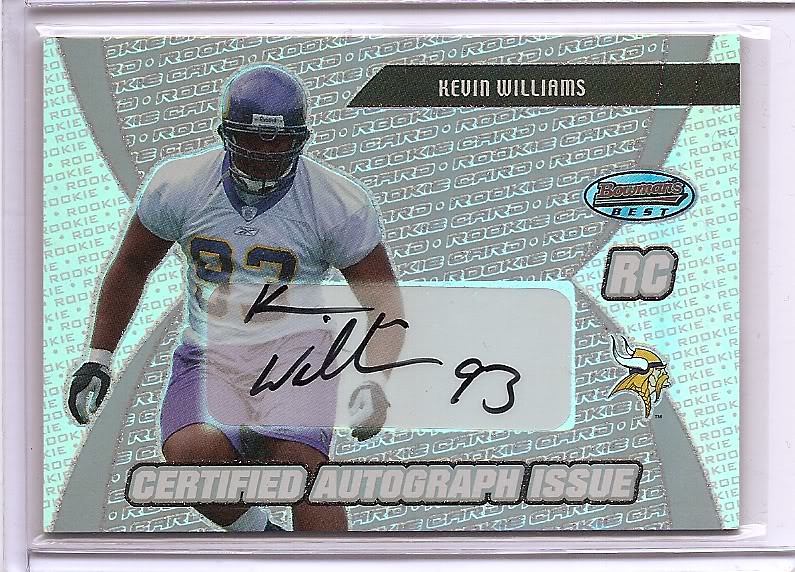This is a detailed image of a Kevin Williams rookie football trading card. The card features a photograph of Kevin Williams, a player for the Minnesota Vikings, captured during practice. He is medium-dark skinned, possibly African American, and is shown in action, running towards the camera with his arms bent at the elbows. He wears a purple helmet with a full face mask, obscuring his face, a Reebok white jersey with the number 93 in yellow and purple, purple shorts, and black and white athletic gloves.

The background of the card is adorned with a repeating pattern of light baby blue and gray geometric shapes. Across the upper right corner, there is a horizontal black bar with a diagonal cut at the center, featuring Kevin Williams’ name in white lettering. Below this bar, there are several logos: an oval logo with the text "Bowman's Best," followed by the initials "RC" indicating it is a rookie card, and a cartoon-style graphic of a Viking with a horned helmet, blonde braid, and mustache—signifying the Minnesota Vikings team logo.

In front of the player image, a white transparent rectangle displays Kevin Williams’ handwritten signature as "K Will 93," signifying it as a certified autograph issue. This autograph is emphasized by the text "Certified Autograph Issue" in white lettering, set on a slightly gray field outlined in black, situated just below the signature. The overall card design prominently marks Kevin Williams' rookie status while showcasing his affiliation with the Minnesota Vikings.